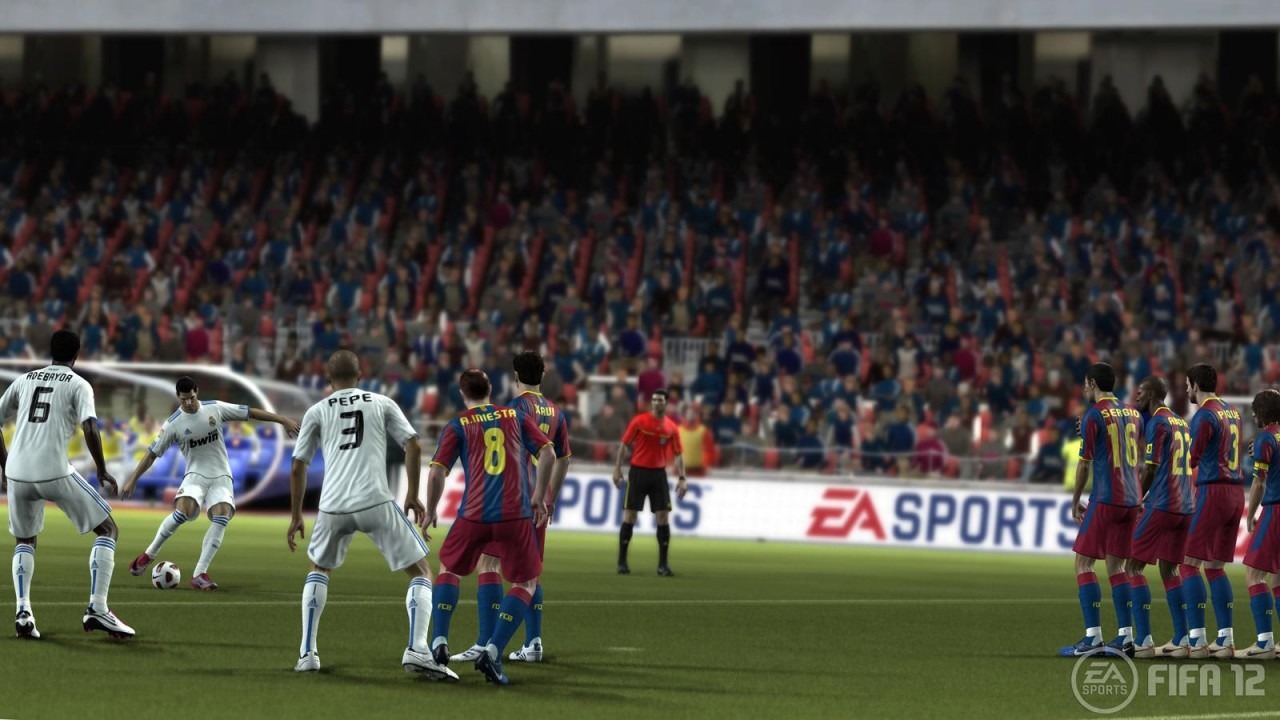The image is a detailed screenshot from the EA Sports video game FIFA 12, depicting a soccer game between Real Madrid and another major club. Real Madrid players are identifiable by their white uniforms with black trim and letters, including knee-length white shorts and white knee socks featuring a blue line. The opposing team wears burgundy shorts, burgundy shirts with blue horizontal stripes, blue socks with burgundy trim, and yellow letters and numbers. The scene captures a pivotal moment where a free kick is being taken from just outside the main box, with players from the burgundy-clad team assembled into a wall formation. A referee, sporting an orange shirt and black shorts, is present on the field. The stadium, filled with spectators, adds to the realistic ambiance, and the prominent EA Sports logo borders the image, underscoring the game's branding.